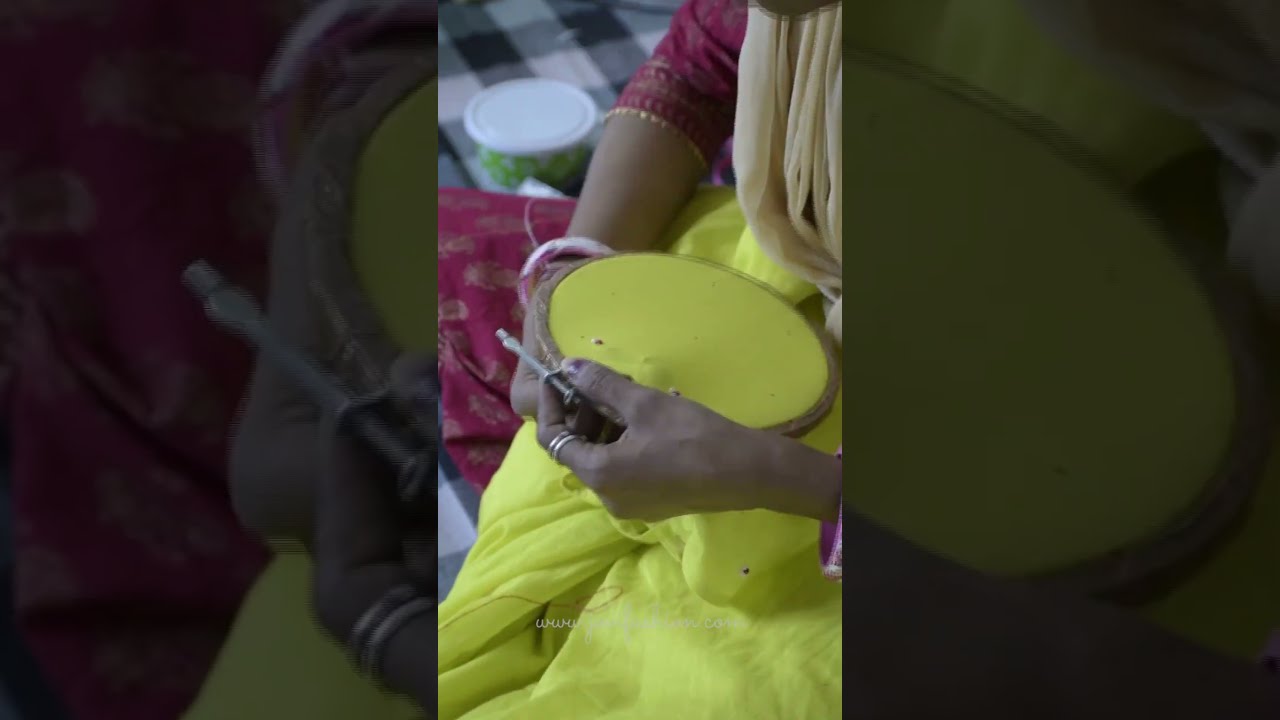The image is a vertically shot screenshot of an instructional video, likely intended for platforms like TikTok. In the center of the image, a woman is engaged in needlework. She is holding a wooden embroidery hoop, likely brown or covered in twine, with a pale yellow cloth secured in it. The woman appears to be preparing to push a needle through the cloth from the underside. She is seated cross-legged on a black, gray, and white plaid blanket. Dressed in a traditional burgundy Indian dress with gold trim and intricate gold patterns, her face is not visible. The woman’s left hand holds the hoop, while her right hand is underneath the fabric, ready to work on it. Nearby, there is a small tub, possibly containing beads, and another container with a white lid and some green contents within, placed at the upper part of the image. The screenshot is bordered by a faded, enlarged, greyed-out section, highlighting the woman and her needlework. Unreadable text is present at the bottom of the image.